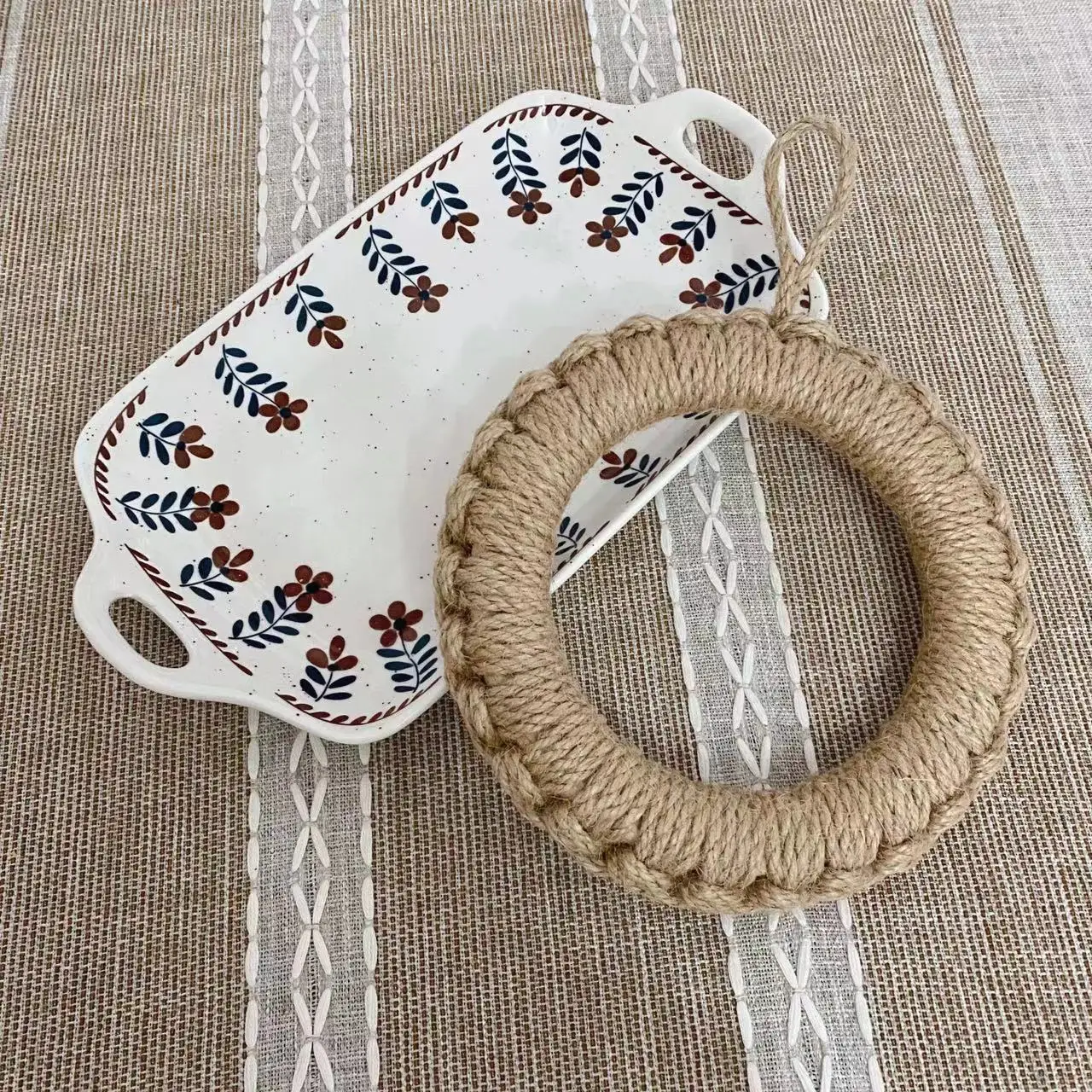The image showcases a square frame featuring two distinct objects centrally positioned on a hessian cloth with intricate vertical and geometric designs. The background is a vertically striped brown hessian with narrow white stitched strips and diamond-shaped patterns reminiscent of a DNA helix running along its length. Dominating the scene is a white rectangular ceramic dish, adorned with handles that have holes for hanging on each side. The dish is embellished with a pattern of flowers, having a bronze base, red or bronze blossoms with black dots in their centers, and greenish-blue leaves, distributed along the edges. Positioned diagonally over the dish and partly resting on the hessian cloth is a woven hessian decoration, possibly a macrame or crocheted wreath. This decorative piece has a loop at the top for hanging and resembles a tightly wound or twined rope, suggestive of a circular dog tug-of-war toy. The overall arrangement highlights the contrast between the rustic texture of the hessian cloth and the delicate, colorful design of the ceramic dish, creating a visually appealing tableau.